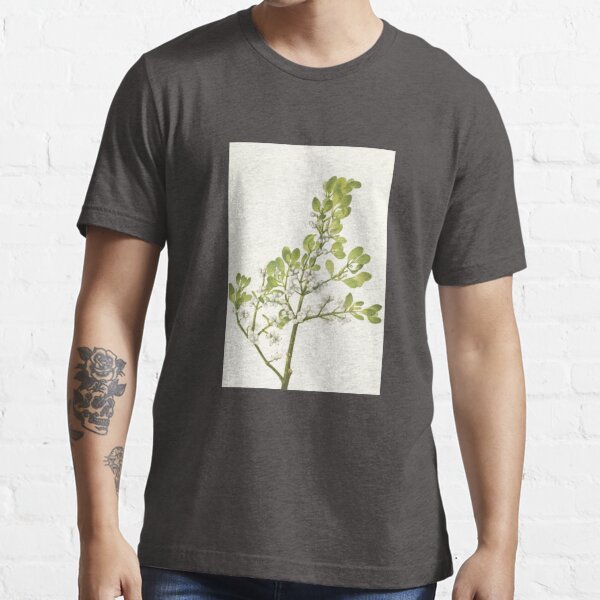This photograph features a light-complected man, head obscured, standing against a white brick wall. The image captures him from the neck to the upper legs. He is attired in a charcoal-colored t-shirt adorned with a distinct white square panel centered on the torso. Within this panel, there's a drawing of a slender tree with sparse branches and green leaves. The man also wears dark denim jeans. Noteworthy are his tattoos: his right arm displays a prominent design featuring a black rose emerging from a skull, while his left arm remains bare. He holds his arms down by his sides.